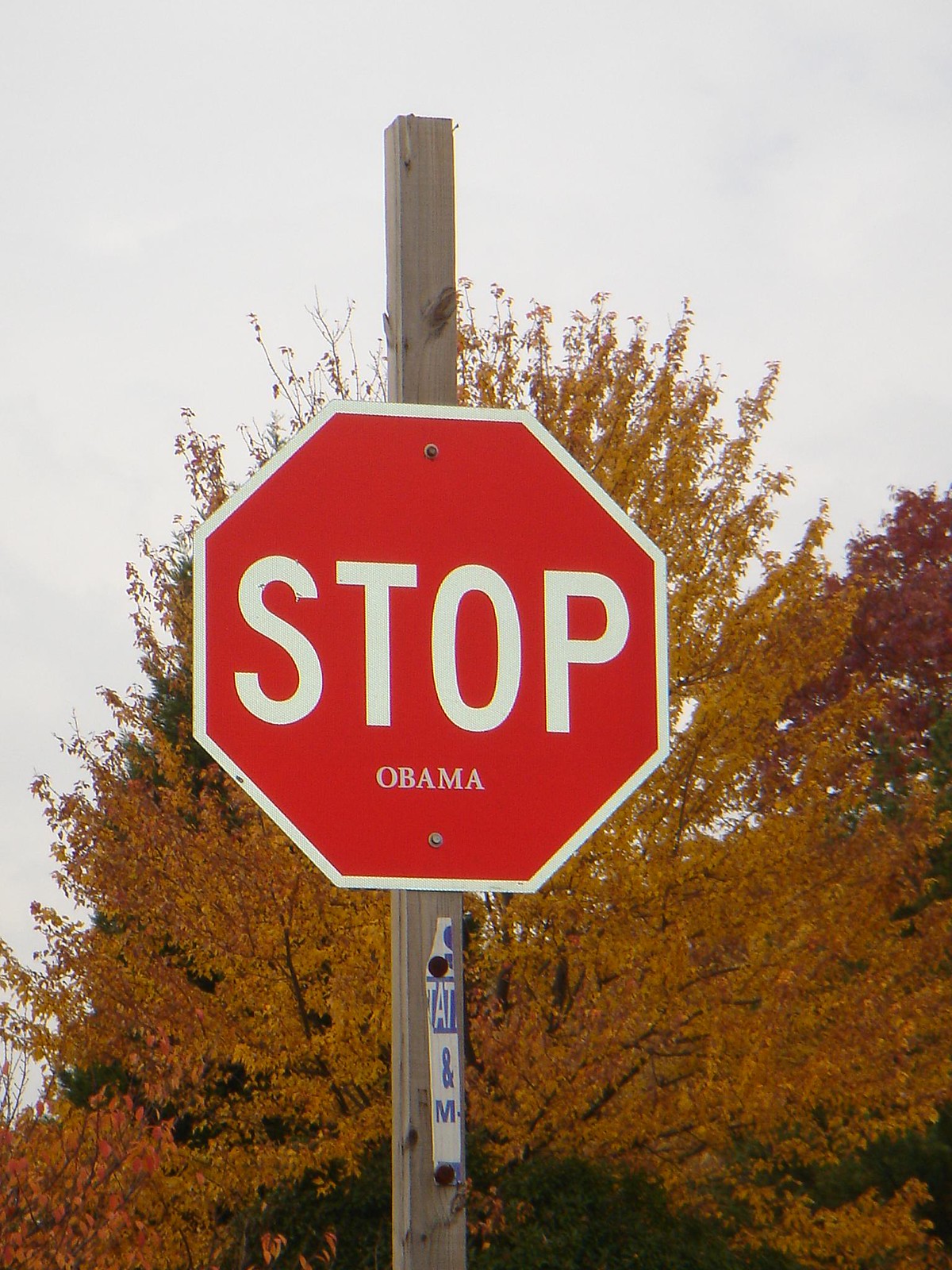This photograph, taken outdoors, captures an autumn scene dominated by a wooden post with a red octagonal stop sign. The sign reads "STOP" in large white reflective letters with a white border around it. Below "STOP," in smaller white letters, the name "OBAMA" has been added. Additionally, a tattered white piece of tape attached to the post bears the partial inscription "T-A-T" followed by an ampersand and the letter "M." The backdrop features a white sky and two mature trees adorned with brownish-yellow, red, and orange leaves, indicative of the fall season. The image composition highlights the foreground with the stop sign and post, while the background of trees is slightly blurred, drawing focus to the sign and its unique additions.